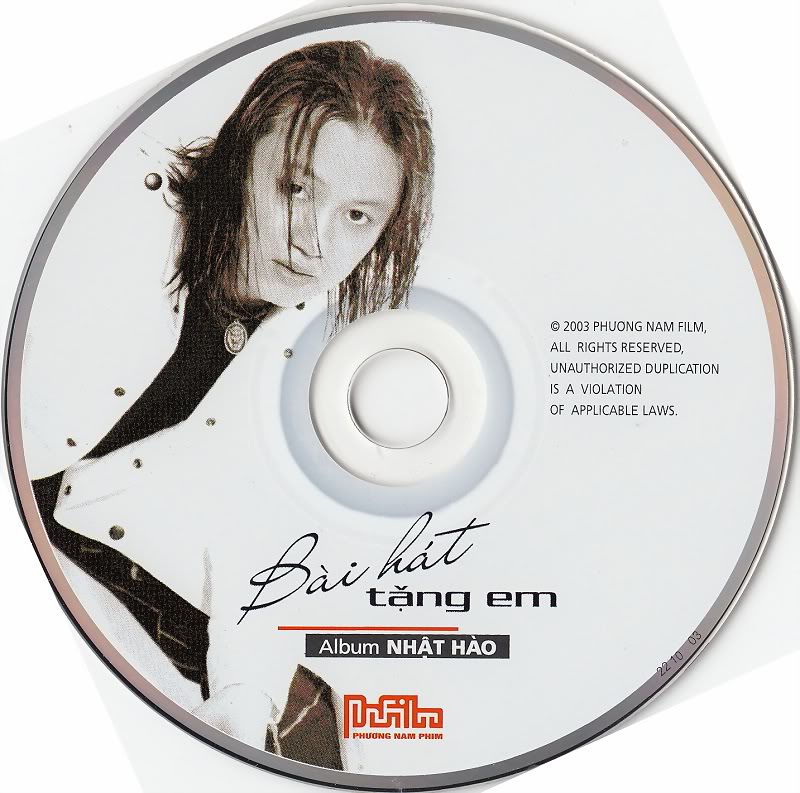This image features a compact disc (CD) positioned against a white background. The CD itself is defined by a silver outer circle that encloses a white surface, with a light gray circle at its core leading into the white plastic inner circle typical of CDs.

On the left side of the CD, the background displays a young clean-shaven Asian male with long, brownish hair that falls to shoulder length, some of it swooshing over his right eye. He is facing the camera directly, possibly bending slightly at the waist. The man is dressed in a white open jacket over a black shirt, accessorized with a silver medallion-type necklace. Only his left arm is visible, as the right arm is cut off by the image boundary, and he is wearing dark-colored pants.

The right side of the CD features text information. At the top, it reads "2023 Phong Nam Film, All Rights Reserved, Unauthorized Duplication is a Violation of Applicable Laws" in black horizontal text. Beneath the center of the CD is the title, which reads "Bài Hát" in a prominent script font. Below this is "Tháng Em" in horizontal text with an accentuated 'a'. A red horizontal line separates this from a black bar, within which "Album Nhật Hào" is inscribed in white lettering. Below the black bar, there is an indistinct red logo, which appears as a squiggled design with unreadable text.